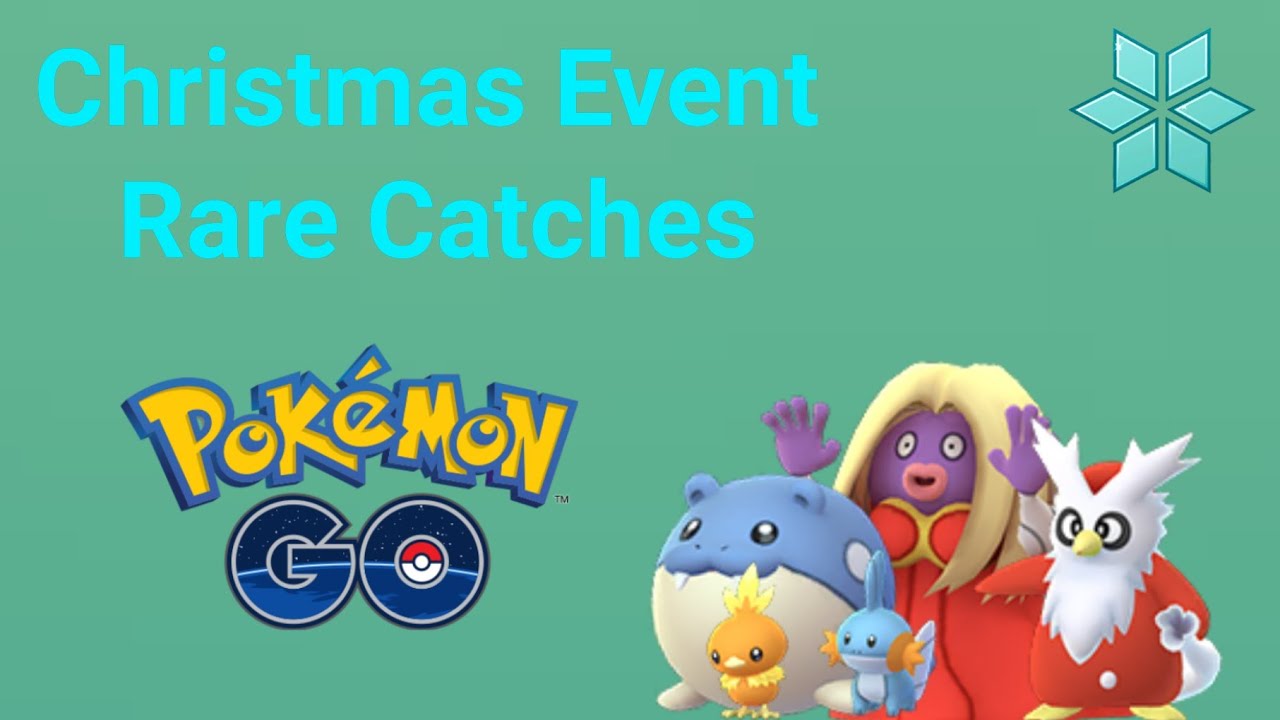The image features a background with a soothing teal greenish hue, overlaid at the top with bold turquoise text that reads "Christmas Event Rare Catches." In the top right corner, there's a striking snowflake symbol composed of six light blue diamond-shaped segments converging at the center. Below this emblem, the iconic yellow Pokémon logo, accentuated with a blue outline around each letter, is prominently displayed. Just beneath it, the word "GO" appears, gradient-shaded from dark purple in the center to light purple on the edges.

The visual is accentuated by a group of Pokémon characters clustered on the right. At the bottom of this assembly is a round Pokémon with a white lower half and a light blue upper head. In front of this figure stands an orange, chicken-like Pokémon. To its right, an owl-like Pokémon character dons a festive red outfit complete with a white beard, yellow beak, and matching yellow feet. The character is further adorned with a fluffy tail, adding a whimsical touch to its appearance.